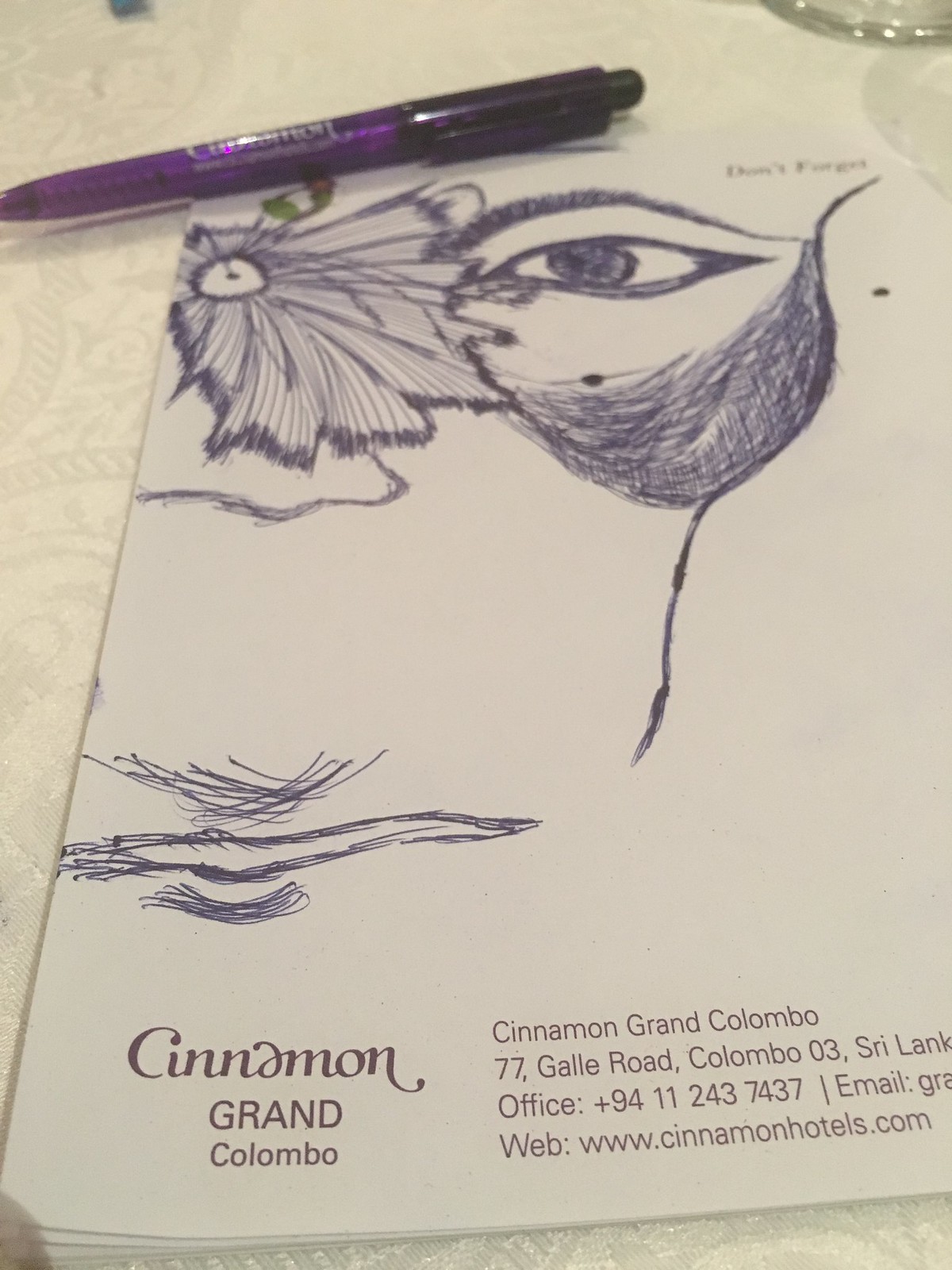An intricate hand-drawn ink illustration on the back cover of a booklet from Cinnamon Grand Colombo captures a fascinating scene. At the top of the drawing, a purple pen rests, indicating the artist’s recent work. The artwork features a possible male face with a pronounced almond-shaped eye extending outward and a slim, refined eyebrow. Below the eye, there is a depiction of a leaf, suggesting nature's intertwining with human elements. The nose is adorned with an open flower, its petals fully bloomed, adding a delicate touch to the composition. Further down, the representation transitions into a symbol resembling a bird. The back end portrays bird-like feet, while the front narrows, reminiscent of certain bird species. Additional minute details scattered across the top and bottom of the drawing likely emphasize and reinforce the bird motif, finalizing this detailed and dynamic illustration.